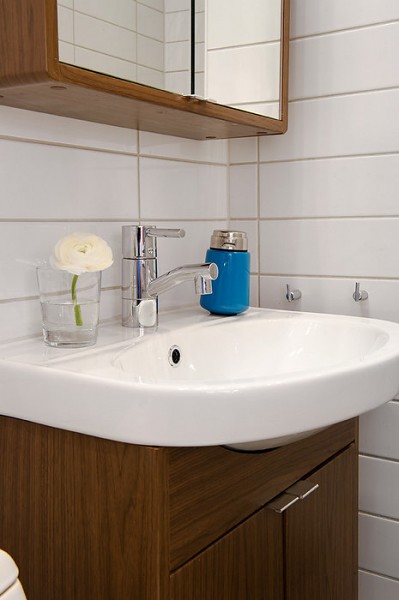In this cozy bathroom corner, the striking elements blend seamlessly to create a polished and inviting space. The white walls, segmented into thirds resembling white boards, provide a crisp, clean backdrop. A brown cabinet with dual doors, adorned with sleek silver handles, anchors the space with a touch of warmth. The large, oval white sink sits atop the cabinet, complemented by the modern silver faucet and controllers designed for effortless operation with a simple up-and-down push.

Peeking from the side is the pristine white toilet, consistent with the room's minimalist aesthetic. Atop the sink, a clear glass vase houses a delicate white rose with a vibrant green stem, partially submerged in water, adding a natural and serene touch. Adjacent to the vase, a metal cup with a blue base and silver top adds a pop of color and functional elegance.

Two small hooks protrude from the wall on the right, perfect for hanging towels or personal items. Above the hooks, a mirrored cabinet with dual reflective panels provides additional storage and depth to the room. This well-curated bathroom corner combines functionality with refined style, making it both practical and visually pleasing.